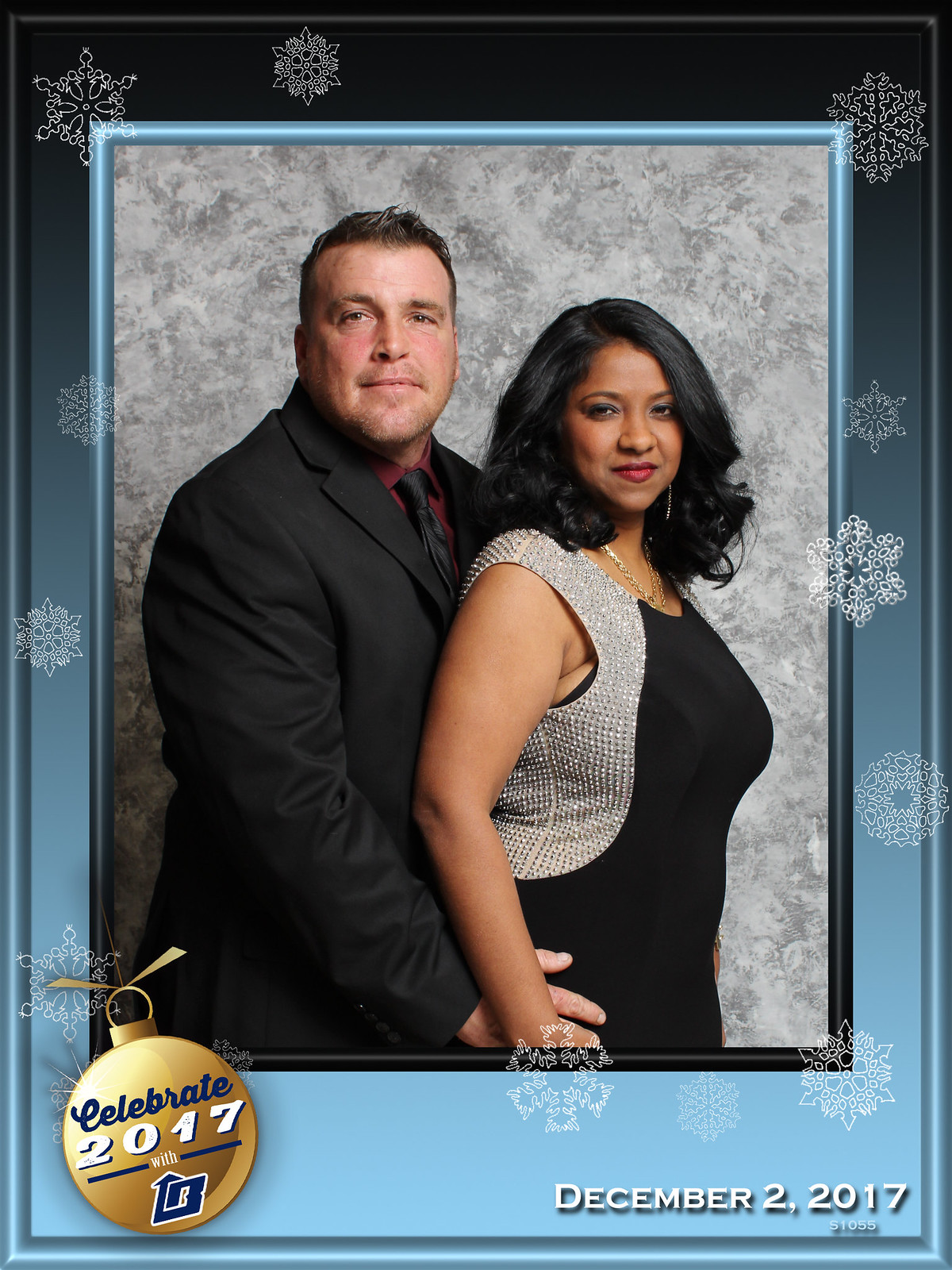In this festive image, Mal, standing to the left, sports short black hair gelled upwards and a matching black blazer, red shirt, and black tie. His broad, neutral face contrasts with his partner’s lively expression. He has white skin and is holding his partner gently by the waist. The woman to his right, with brown skin and cascading black hair curled at the ends, wears pink lipstick and is dressed in an elegant black and silver dress, highlighted with silver around the arms and on the sides. She accessorizes with gold jewelry around her neck and ears. They pose against a gradient background that transitions from black to blue, surrounded by a light grey border adorned with white snowflakes, creating a Christmas card effect.

The card is framed by a blue border, with a golden bauble in the bottom left corner that reads "Celebrate 2017" in blue and white text. A white capitalized "B" icon appears, and "December 2, 2017" is inscribed on the bottom right in white. The image beautifully captures the couple on a special occasion, set against a backdrop evoking a winter wonderland.